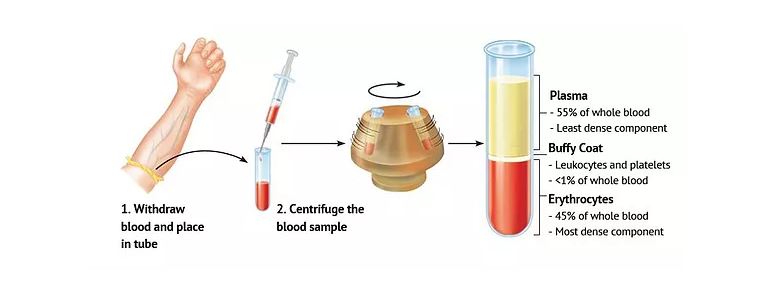The image is a detailed, step-by-step graphic illustration of the blood processing procedure. The process begins on the left with an image of a donor's arm, showing prominent veins due to a tourniquet. Below this, the caption instructs to "withdraw blood and place in tube." An arrow leads to the next image where a syringe is shown depositing blood into a collection tube, accompanied by the text "centrifuge the blood sample." The sequence continues with an image of a centrifuge in operation, indicated by a circular arrow, reflecting high-speed spinning. The final part of the illustration shows the resultant layers within the test tube: the top layer is labeled as "plasma, 55% of whole blood, least dense component," the middle layer, known as the Buffy Coat, contains "leukocytes and platelets, less than 1% of whole blood," and the bottom layer consists of "erythrocytes, 45% of whole blood, most dense component." The graphic uses colors such as blue, white, and red, along with flesh tones to represent these components accurately.